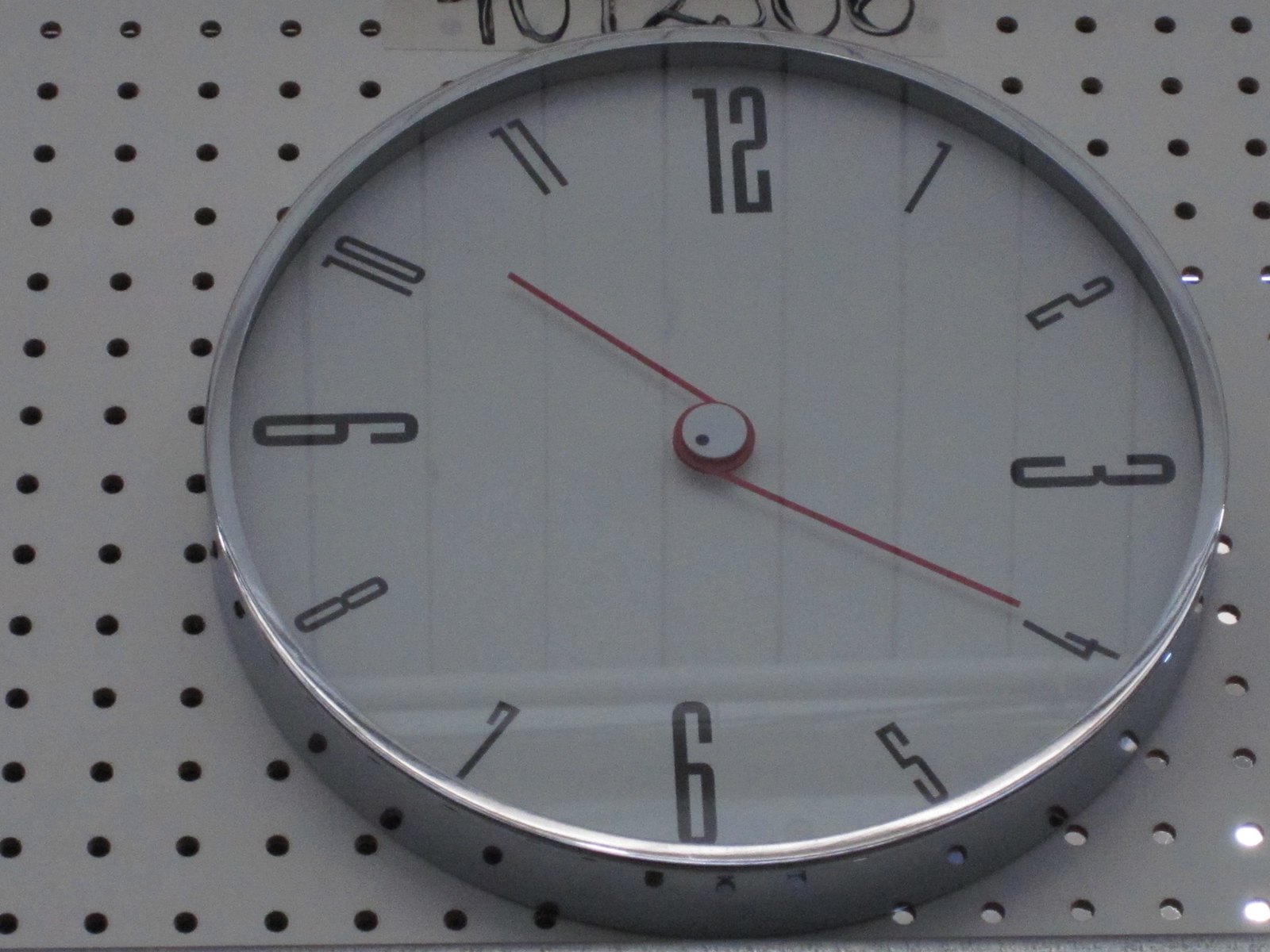An image features a sleek clock mounted on a white pegboard. The clock displays the time as approximately 10:20. Its thin, delicate red minute and hour hands stand out against the white clock face. Prominently, the numbers 12, 3, 6, and 9 are larger than the other numerals, making them easily readable. Encasing the clock is a refined silver rim that adds a touch of elegance to its design. A mild reflection is visible on the clock's glass surface, showing a blurred image of a wall. Above the clock hangs a piece of paper with some numbers, although they are too indistinct to be deciphered.